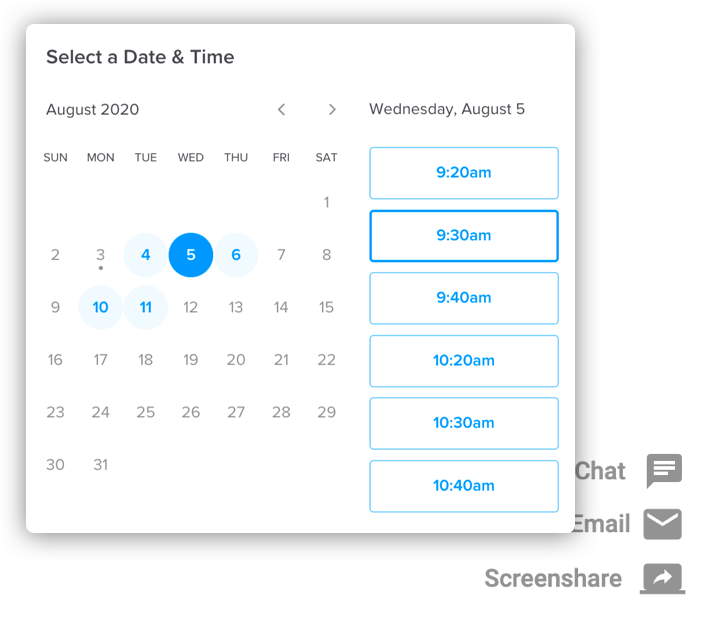The image depicts an onscreen calendar interface, displaying two layers: a mostly obscured background page and a prominent foreground dialog box. The background appears to include options for "Chat," "Email," and "Screen Share" located at the bottom right corner. The foreground dialog presents a calendar review for August 2020, currently focused on August 5th. An event is scheduled at 9:30 AM, but specific details are not visible.

Distinctive color coding is used: the current date, August 5th, has a blue background, while adjacent dates such as the 4th, 6th, 10th, and 11th are highlighted in a light blue shade. August 3rd shows evidence of a past event. The interface includes navigation arrows likely for shifting between months or years, and displays various time slots throughout the day, such as 9:40 AM, 10:20 AM, 10:30 AM, and 10:40 AM, potentially for appointment scheduling. The overall background is white, making the highlighted dates stand out for easy reference.